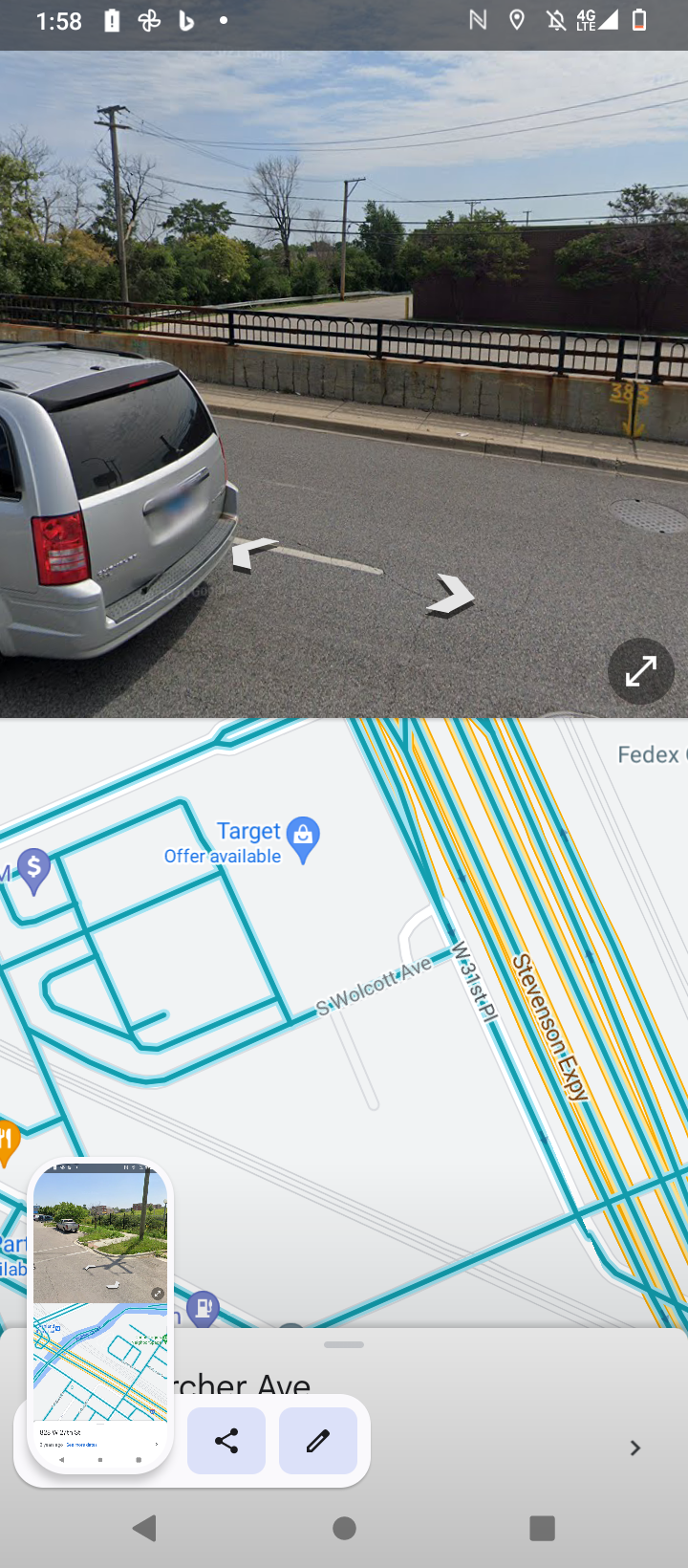The screenshot captures a detailed view of a phone screen. At the top, the time displayed is 1:58 PM, accompanied by several status icons indicating, among other things, that the battery is low. The upper section of the screen features a real-life view of a street, showcasing the rear of a gray vehicle. Adjacent to the street are a sidewalk and a gate, with pavement, trees, and a brown commercial building in the background. In the bottom portion of the screen, a map is visible, highlighting the Stevenson Expressway and a marker indicating an offer available near a Target store. Additionally, there’s a small icon resembling a phone that displays a similar view, with the upper half showing a real-life street and the bottom part replicating the map.